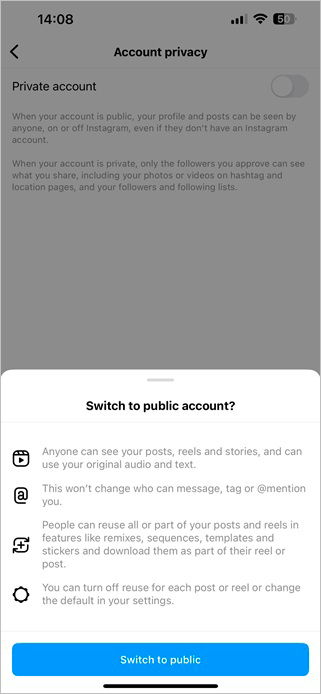The image showcases a screenshot, set against a gray background, with various interface elements reflecting a device's status and an app's settings. The top of the screen displays the current time, 14:08, in bold black text at the upper left corner. In the top right corner, icons denote device connectivity and battery status, showing three out of four Wi-Fi bars, active Wi-Fi, and a battery level at 50%.

Below this status bar, centered in bold black text is the heading “Account Privacy.” To the left side of this heading is a left-pointing arrow. Directly underneath, “Private Account” is written in bold text followed by a toggle button on the right side, which is currently switched off. 

The accompanying descriptive text elaborates: "When your account is public, your profile and posts can be seen by anyone on or off Instagram, even if they don't have an Instagram account. When your account is private, only the followers you approve can see what you share, including your photos or videos on hashtag and location pages, and your followers and following lists."

Towards the bottom of the screenshot, a pull-up page stands out in a white background with the option to "Switch to Public Account" written in bold black text.